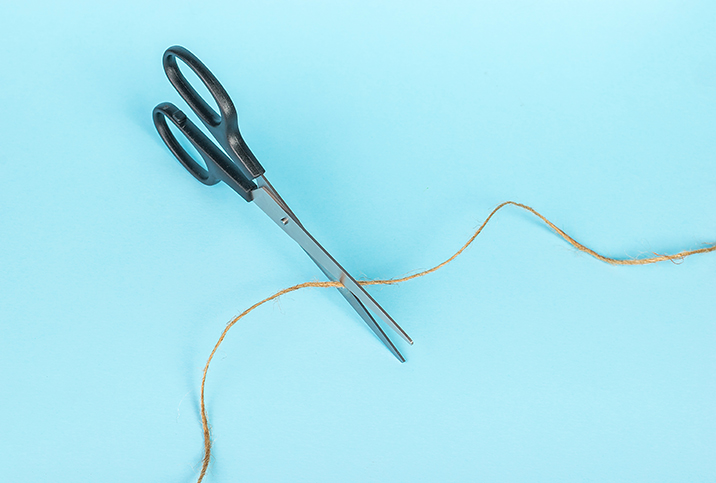This image showcases a detailed scene of a long, slim pair of scissors poised to cut a piece of tan, curly twine. The scissors, featuring silver blades and black handles, dominate the composition with the handles positioned towards the upper left corner and the blades extending to the center. The twine, a beige string, weaves its way from the center right, curving and dropping to the bottom third from the right. The scene is set against a light turquoise blue background, evoking a Tiffany's blue hue. The scissors are slightly open with the twine nestled between the blades, indicating that the cut is just about to commence, yet the twine remains intact. There is no person visible in the image, allowing full focus on the imminent action of the scissors cutting the twine.